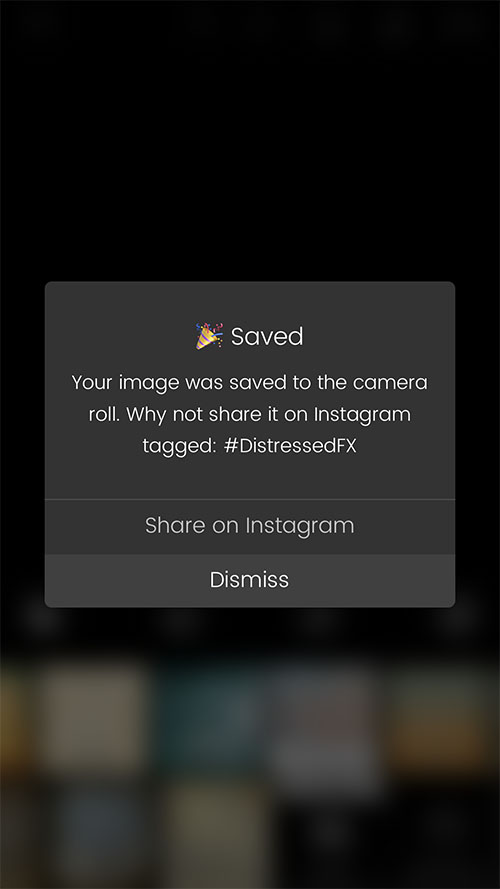The image depicts a mobile device screen displaying a notification. The upper part of the screen features a black background, while the lower half is dominated by a blurry image composed of indistinct squares. Centrally superimposed over the blurry section is a grey rectangle containing several lines of text. At the top of this rectangle, the word "Saved" appears prominently in large white font, accompanied by a small celebratory icon. Below this, a message in white lettering reads, "Your image was saved to the camera roll. Why not share it on Instagram tagged #distressedFX?"

A thin grey line separates this message from the following options. Underneath this line, a heading reads "Share on Instagram." Below this, a slightly lighter grey panel features the option "Dismiss" in white font. The user is prompted to either share the saved image on Instagram or dismiss the notification.